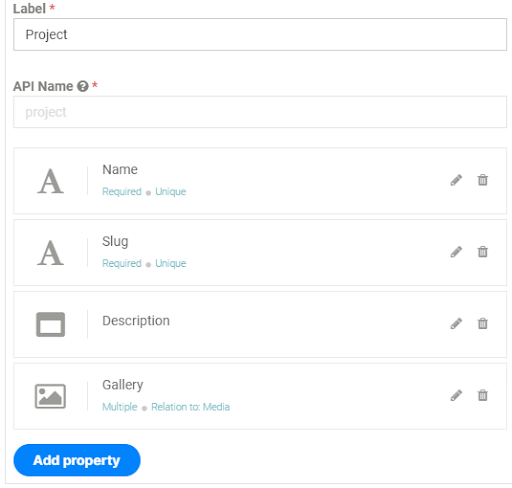In this image, the background is solid white, adorned with very small light blue lines. At the top of the image, there is a light gray label that includes a small red asterisk next to it. Below this, there is a box labeled "Project," followed by another entry labeled "API Name" that features a gray circle with a white question mark inside and another red asterisk beside it.

Continuing downward, there is a section with a large "A" and the word "name" highlighted, with the terms "request" and "unique" joined by a dot. To the right of this text, there are icons of a pencil and a trash can. Below this, another line features a large "A" and the word "slug," similarly accompanied by the terms "required" and "unique" with a dot between them, and again, there are pencil and trash can icons to the right.

The next section includes a box labeled "Descriptions," also accompanied by pencil and trash can icons. Further down, there is a "Gallery" label, also paired with the pencil and trash can icons. Finally, at the bottom of the image, there's a prominent blue button labeled "Add Property."